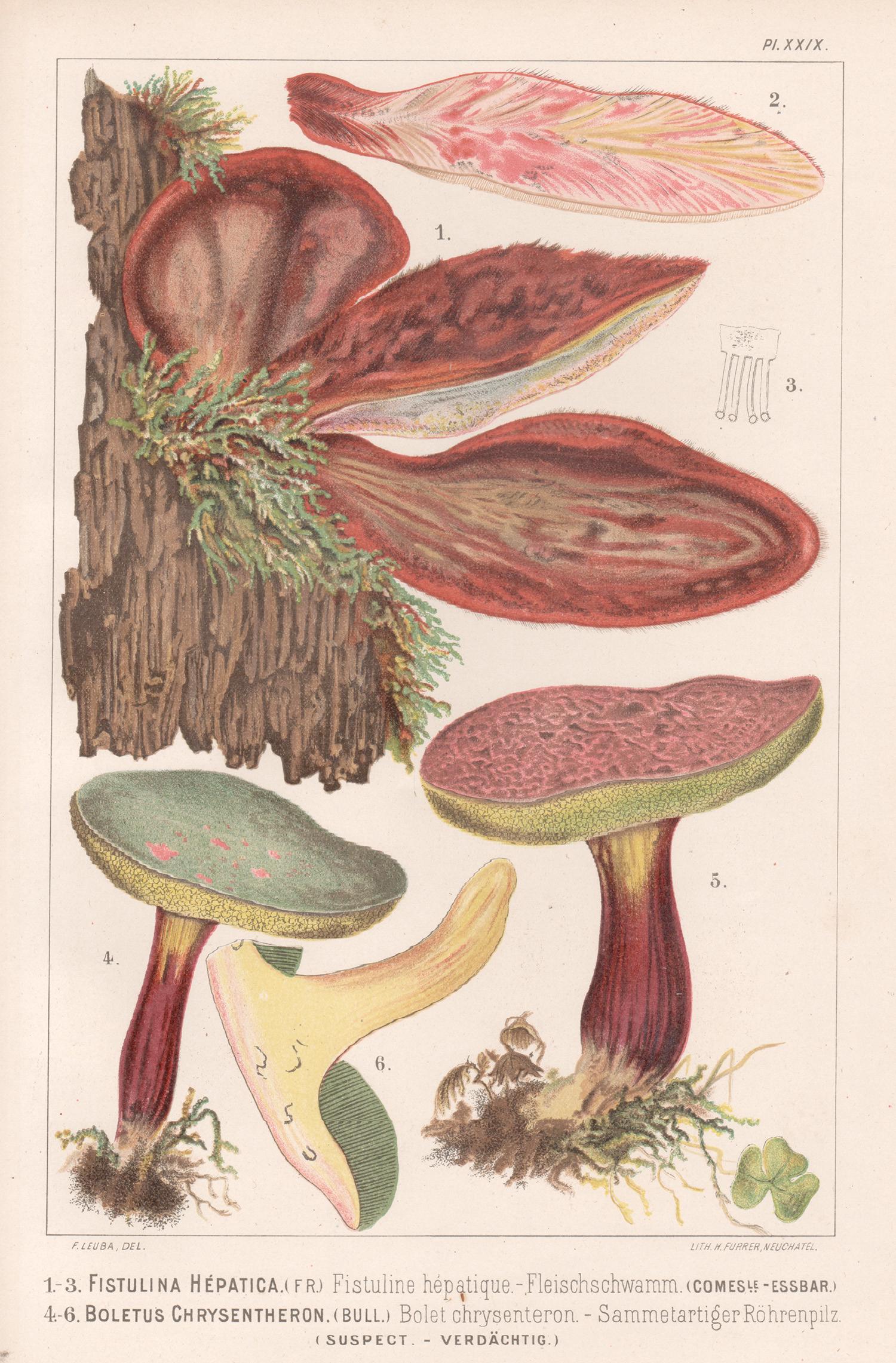The image is a vertically aligned rectangular illustration resembling a page or a poster with a very light brown background, stained slightly in the lower left corner with a gray spot. It is bordered by a thin black line on all sides. Dominating the center are detailed drawings of mushrooms, each labeled with numbers one through six. 

In the lower left, mushroom number four has a brown stem with a green round cap adorned with a couple of brown spots. Next to it, mushroom number six, is positioned with its stem pointed upward. Along the bottom right, mushroom number five features a thick brown stem supporting a textured coral and brown cap.

The upper left section of the image showcases number one, which appears to be growing out of brown wood bark accompanied by green weeds or leaves, with three distinct brown mushrooms sprouting from it. In contrast, the upper right corner holds number two, which resembles a leaf shape with a brown base that transitions into coral, pink, and yellow tips.

The mushrooms are illustrated in a range of colors including burgundy pink, tan, purple with an olive green border, and seafoam green with a gold border. The identifying labels spell out "Fistulina hepatica" for mushrooms numbered one through three, and "Boletus chrysenteron" for mushrooms four through six.